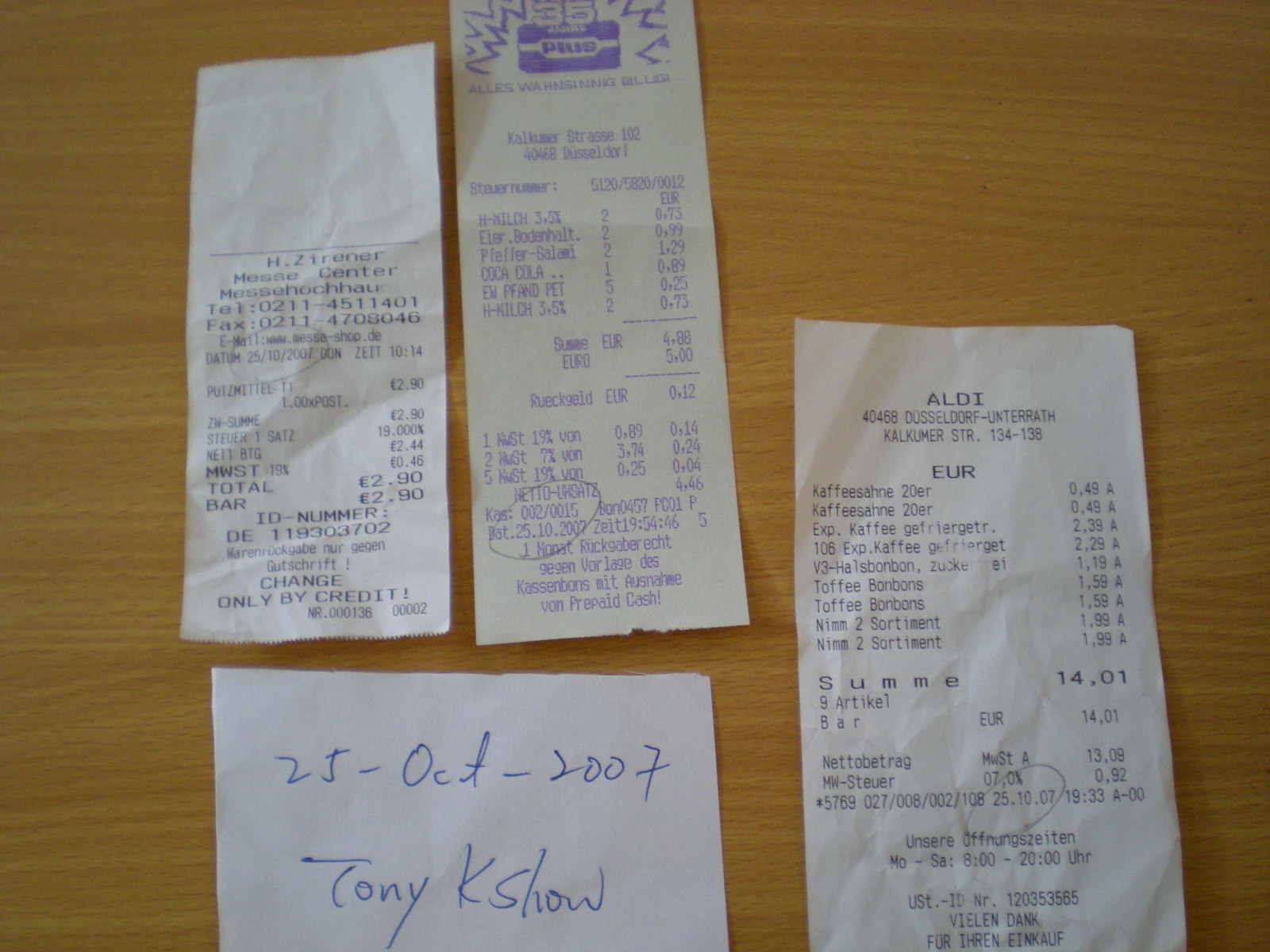The image captures a close-up of five white pieces of paper arranged on a light brown wooden tabletop. Prominently, there are three store receipts with details written in varying text colors, including black and purple, and several dates circled. To the left, a receipt features a message center from "HZ Treanor," while above it, another receipt with blue typing displays the date 25-10-2002. The rightmost receipt is from ALDI, showcasing a total amount of €14.01, and has the date 25-10-07 circled. At the bottom of the image lies a slightly crumpled white piece of paper, bearing the handwritten date 25 October 2007 and the name Tony K. Cho written conspicuously in blue ink.